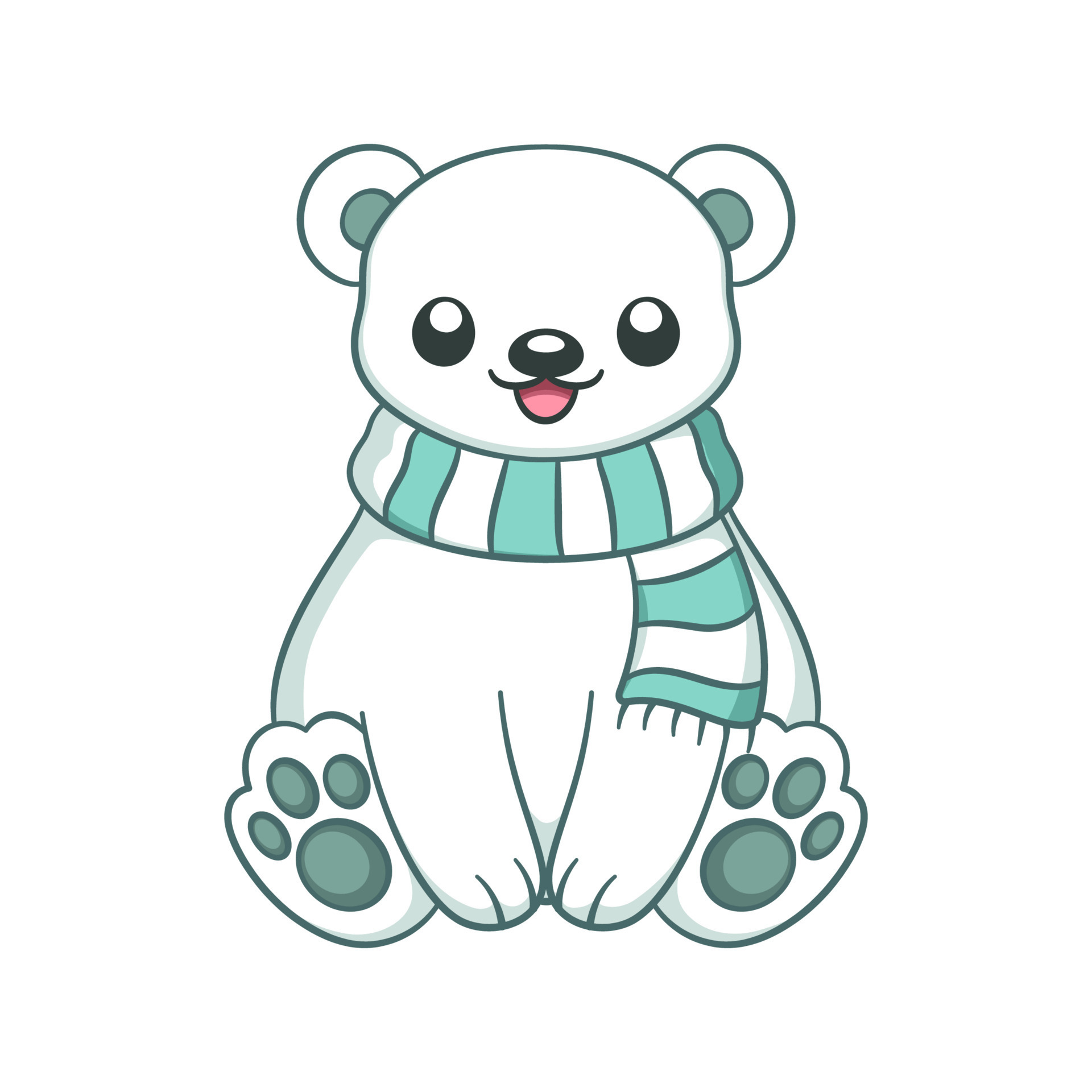This is a detailed, cartoon-style image of a smiling polar bear cub sitting upright on a completely white background. The bear's design includes various shades of white and green. It wears a green and white striped scarf around its neck, and has greenish-blue inner ears and paw pads. The bear is positioned with its front paws resting on the ground between its back legs, facing the viewer directly. The image also features the bear's mouth open in a grin, revealing a hint of its pink tongue. It is a clean and simple illustration with no other elements in the background, emphasizing the cute and charming nature of the polar bear cub.